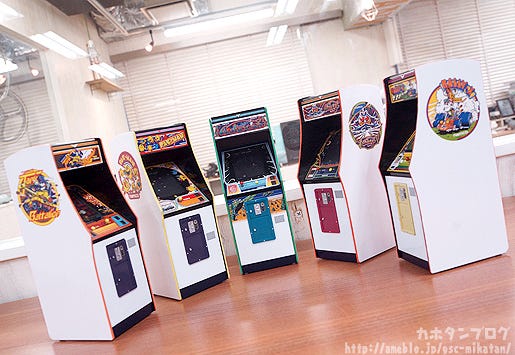The image depicts five vintage arcade machines from the 1970s and 1980s, arranged in a semicircle on a wooden floor. The white arcade cabinets feature colorful front plates for the coin slots, which come in purple, blue, red, and beige colors. The machines have black interiors where the screens and controls are located, along with multicolored symbols and labels on the tops and sides that are hard to read clearly. Notably, one of the machines appears to be a Pac-Man game. The photo was taken at an angle, revealing a modern office environment in the background, characterized by contemporary lighting, white blinds, and HVAC equipment. In the lower right-hand corner, Japanese characters and symbols are visible, suggesting the popularity or origin of these games in Japan.